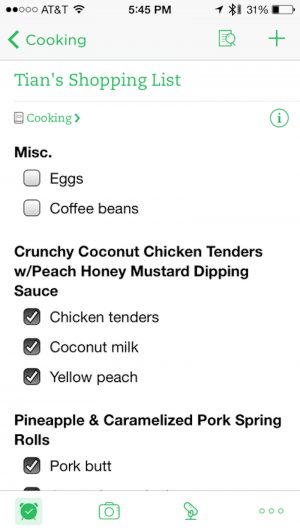This mobile screenshot captures the "Shopping List" page from a cooking app. At the top left, the word "Cooking" is prominently displayed in green, accompanied by a left-pointing green arrow. On the top right, there is an icon of a piece of paper with a magnifying glass overlay, suggesting a search function for the page, and a plus sign positioned further to the right.

Below this header, the title "Tian's Shopping List" is displayed in large green letters. Beneath this, the word "Cooking" reappears with another left-pointing arrow. The screen is divided into categories, each with associated checkboxes.

The first category, labeled "Miscellaneous," includes two items: eggs and coffee beans, both with unchecked checkboxes. The second category is "Crunchy Coconut Chicken Tenders with Peach Honey Mustard Dipping Sauce." Under this, the items listed are chicken tenders, coconut milk, and yellow peach, all marked with clip icons, indicating they are selected.

At the very bottom of the screenshot is the category "Pineapple and Caramelized Pork Spring Rolls," showing pork butt, which is clipped, with another checkbox partially cut off from the screen's body.